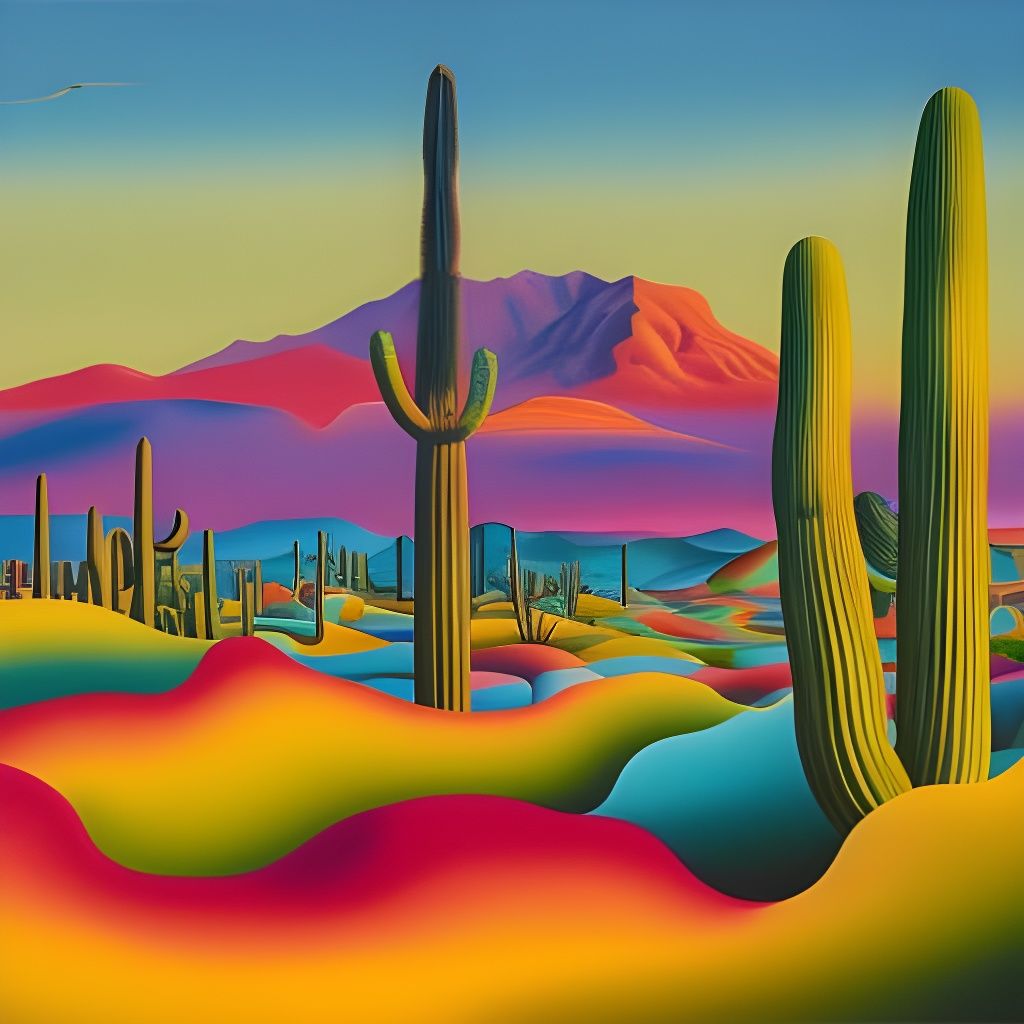This vibrant, psychedelic 3D graphic image portrays a surreal desert landscape under a dynamic sky. The sky transitions from deep blue at the top to a greenish lime and gradually turns yellow, filling the scene with a sense of motion and color shift. Dominating the foreground are large, dark green cacti, including one central light green cactus that darkens towards its top. These cacti stretch from the rolling, wavy, sand-like ground—where colors blend into waves of red, yellow, and green—towards the upper part of the image.

In the background, a dramatic mountain range catches the eye with its striking hues. The right side of the mountains is an intense orange that fades into blue and purple in the center. As the ridge moves left, it becomes red, juxtaposed beneath an intermediate purple and light teal section. The base of the mountains, interspersed with additional blue, blends into the colorful landscape, creating an almost thermal visual effect. This distinctive combination of shifting colors and organic shapes results in a mesmerizing desert scene, far removed from traditional depictions, evoking a sense of otherworldly beauty.